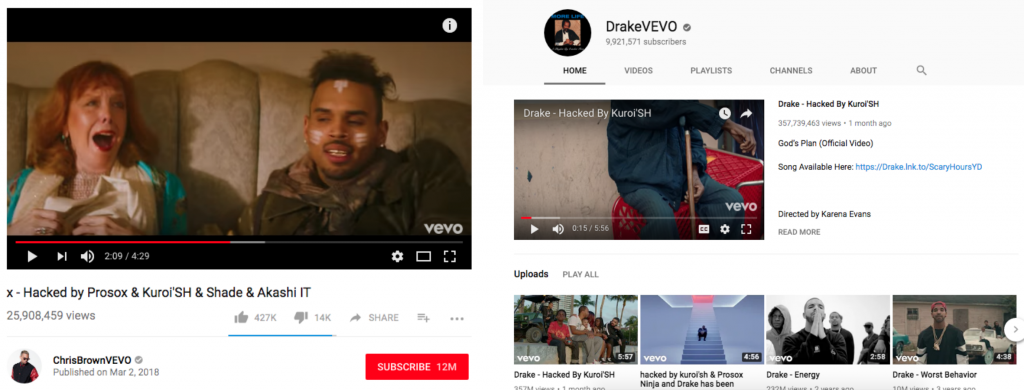This caption reflects a detailed analysis of two side-by-side YouTube screen grabs featuring content from VEVO channels.

---

The image displays two YouTube screen grabs placed side by side. The first screen grab appears to showcase a music video, possibly titled "Moose Music Video." It features a Caucasian red-haired woman wearing red lipstick and a turquoise coat, and a brown-skinned man dressed in a brown coat with white paint on his face. Both are seated on a tan, floral-patterned couch. The VEVO watermark is visible in the corner alongside various icons, including a play button, speaker icon, settings cogwheel, rectangle, and square icons. The video shows 209 out of 429 seconds elapsed. The title in black text reads "X hacked by Prosox and Kuroi'SH," with a view count of 25,908,459. The video has garnered 427,000 thumbs up and 14,000 thumbs down. Additional details indicate that this content is from the Chris Brown VEVO channel, published on March 2, 2018, with a red subscribe button on display.

On the other side, the second screen grab is from the Drake VEVO channel, which boasts 9,921,571 subscribers. The top section features menu options, such as home, videos, playlist, and channels, laid out against a white background with gray, blue, and black fonts. Below these headers is a snapshot of a video titled "Drake hacked by Kuroi'SH." The image depicts a person dressed in navy blue sitting atop a red shopping cart against a tan wall. The play counter indicates that the video is "God's Plan Official Video," directed by Karena Evans. Moreover, the video's description includes a URL. Beneath this, a series of related images preview other videos titled "Drake hacked by Kuroi'SH," "Drake Energy," and "Drake Horse Behavior." These thumbnails show various scenes: people sitting on concrete, people on blue stairs, individuals in black and white, and a man with darker skin wearing a black shirt and gold necklace standing by some cars. 

---